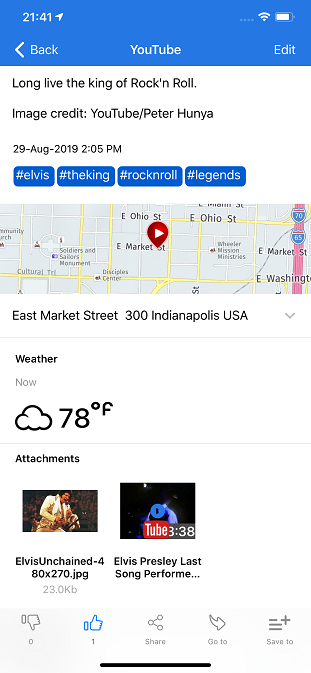A nostalgic glimpse into the past: This image captures an old version of the YouTube app, showcasing a tribute to Elvis Presley with the caption, "Long live the king of rock and roll." The image credit goes to Peter Hania. The post is adorned with several hashtags: #Elvis, #TheKing, #RockAndRoll, and #Legends. A small map pinpoints a location at East Market Street, 300 Indianapolis, USA, suggesting the site could be associated with an Elvis cover artist or a commemorative event.

On the screen, the current weather reads 78 degrees Fahrenheit with cloudy conditions. Attached to the post, there's a nostalgic black-and-white photo of Elvis from his “Elvis Unchained” performance, alongside a link to a video titled "Elvis Presley's Last Song Performance." At the bottom of the screen, user interaction buttons include thumbs up, thumbs down, share, and save options, all set against a white background accentuated with various blue elements.